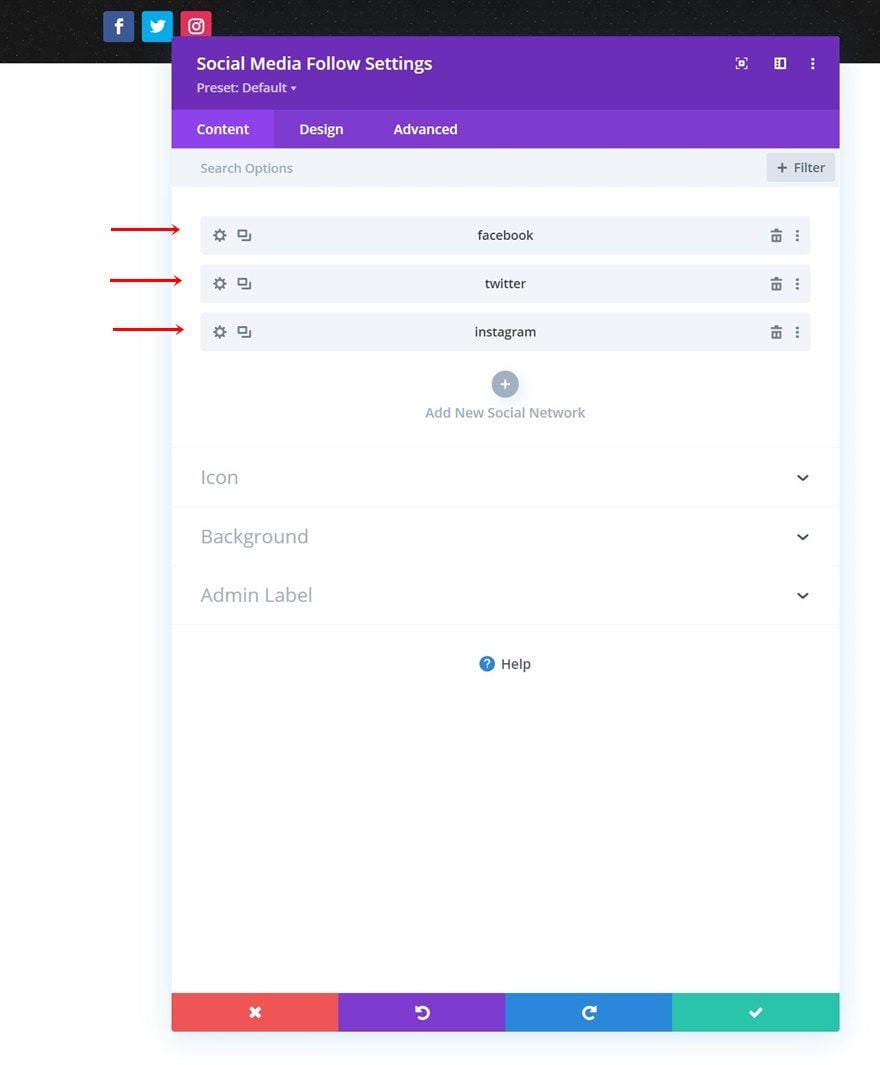The image is a detailed screenshot of a social media settings interface, likely for a web or mobile application. At the top of the screenshot, there is a black horizontal bar containing links represented by the Facebook, Twitter, and Instagram logos. 

Superimposed in front of this bar is a smaller square with the heading "Social Media Follow Settings" and a preset option labeled "default." A dropdown menu is available for changing this preset, and this section is highlighted with a purple banner.

Below the purple banner are three tabs labeled "Content," "Design," and "Advanced," with "Content" being the currently selected tab. This section provides various options, including "Search Options" and "Filter."

Following this, there are individual columns for Facebook, Twitter, and Instagram, each marked with a red arrow pointing at them from the left. Each social media column contains its own settings tool and trash can icon for managing the options.

Further down, there is an "Add New Social Network" option accompanied by a plus sign within a circle. Below this, three dropdown menus are labeled "Icon," "Background," and "Admin Label."

A help button with a hover effect is centered below these dropdown menus. Finally, at the bottom of the screenshot, there are four clickable buttons in different colors: a red 'X', a purple reload icon, a blue reload icon, and a green check mark.